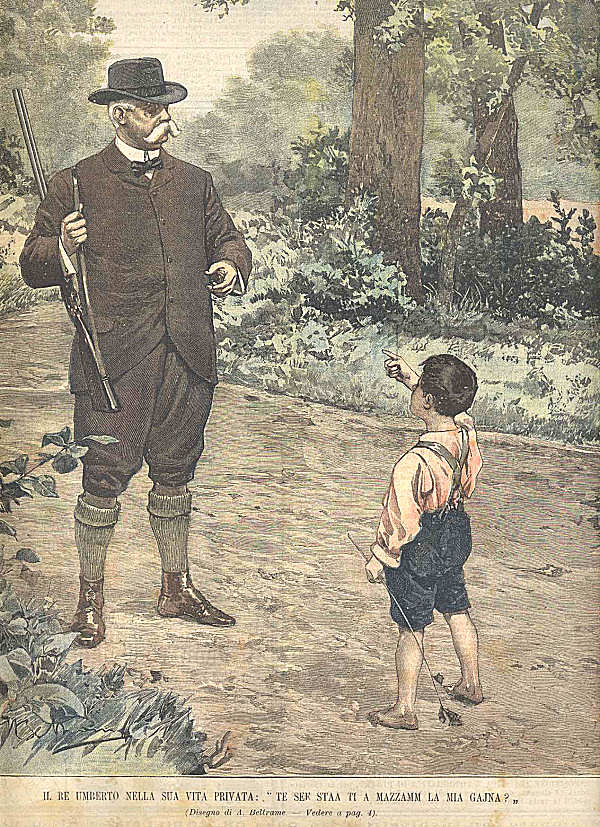The image resembles a photorealistic drawing or painting from an old magazine or newspaper, showcasing remarkable attention to detail. Central to the image is an older man, bearing a striking resemblance to Theodore Roosevelt, dressed in a brown suit with his pants rolled up to reveal knee-high socks. He sports a brimmed hat and a bushy white mustache, and carries a double-barrel shotgun slung over his shoulder. He is positioned slightly to the left, gazing to the right. Beside him on a woodsy path stands a barefoot boy in black shorts, suspenders, and a reddish button-up shirt, pointing up at the man. The background features a woodland setting with trees, bushes, and a glimpse of the sky. At the bottom of the image, there is non-English text, including the caption "RE Umberto Nella SUA VITA PRIVATA," and additional notes that appear to describe the scene or provide context.